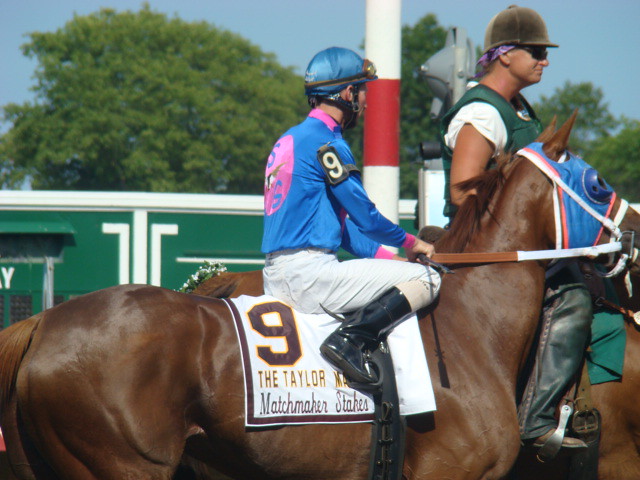This vibrant outdoor photograph captures a dynamic moment at the horse racing track, featuring a side view of a brown horse adorned with a blue hood and blue blinders, prominently marked with a white banner displaying the number nine. The banner partially reads "The Tailor Matchmaker Stakes." Seated atop the horse is a jockey, dressed in white pants and tall black boots, with his feet firmly in the stirrups. The jockey wears a blue shirt with a pink collar and a matching blue helmet, complemented by a pink and blue emblem on the back. The number nine is also visible on his right sleeve. In the background, there is a man in a brown cap, a white t-shirt, and a green vest, standing next to the horse. The setting is bright and outdoors, with a clear blue sky, trees, and a green building with white trim and a green awning providing the backdrop. A partially visible second horse and jockey are obstructed by the prominent brown horse in the foreground.